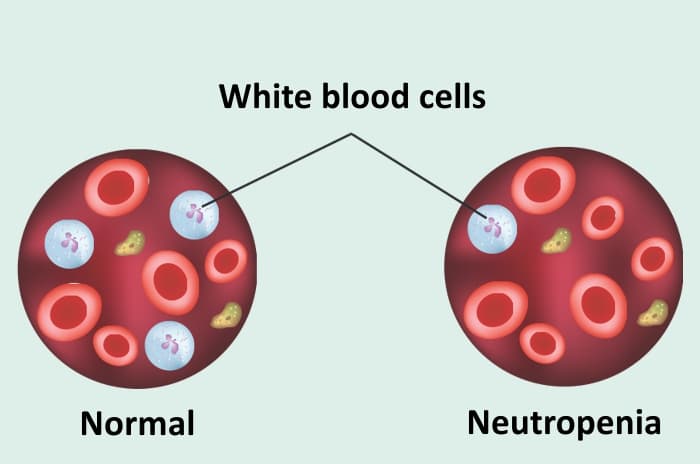This infographic features an illustration with a pale pink background, entitled "White Blood Cells" in prominent black letters at the top. Two side-by-side circular depictions visualize the differences in white blood cells. On the left, labeled "Normal," the illustration shows a typical blood sample with three white blood cells, identifiable by their white circles containing purplish dots, and surrounded by fewer red blood cells—pink rings with dark red centers. On the right, labeled "Neutropenia," the image displays a blood sample reflecting neutropenia, characterized by a significant decrease in white blood cells—showing only one white blood cell amidst a greater number of red blood cells. This comparative visual effectively highlights the contrast between a normal blood cell composition and one affected by neutropenia, showcasing fewer white blood cells and a higher proportion of red blood cells in the latter.